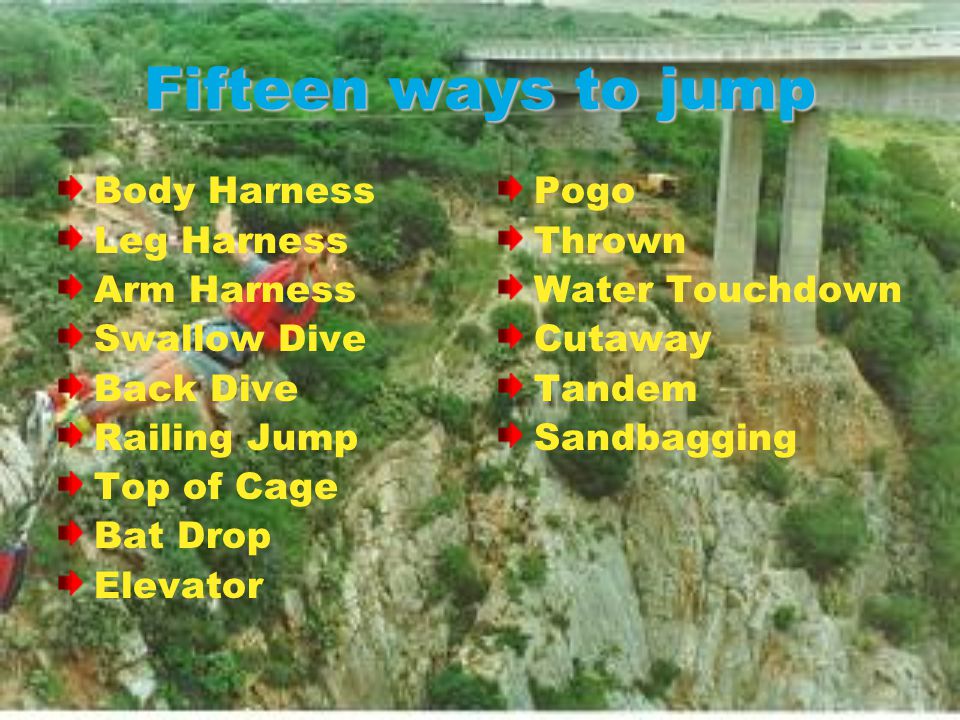The image is an old advertisement card for bungee jumping, characterized by a scenic background and detailed instructions. The main visual focus is a person in light-colored shorts, a red harness vest, with long blonde hair, captured in mid-air as they dive off a rocky ledge, possibly performing a form of cliff diving or bungee jumping. Their arms are spread wide, emphasizing the sense of flight. The backdrop features a picturesque hillside with interspersed grass and trees. Prominently visible on the right side is a bridge supported by two substantial concrete buttresses, stretching from the upper right to the left and partially obscured by the treeline. The top of the card boldly displays the title "15 Ways to Jump" in blue letters, while the left side and then a section further to the right lists methods for jumping, framed by red arrows pointing to yellow text. These methods include: Body Harness, Leg Harness, Arm Harness, Swallow Dive, Back Dive, Railing Jump, Top of Cage, Bat Drop, Elevator, Pogo, Thrown, Water, Touchdown, Cutaway, Tandem, and Sandbagging. The card, though outdated, vividly conveys the adventurous spirit of bungee jumping through its detailed depiction and instructional content.